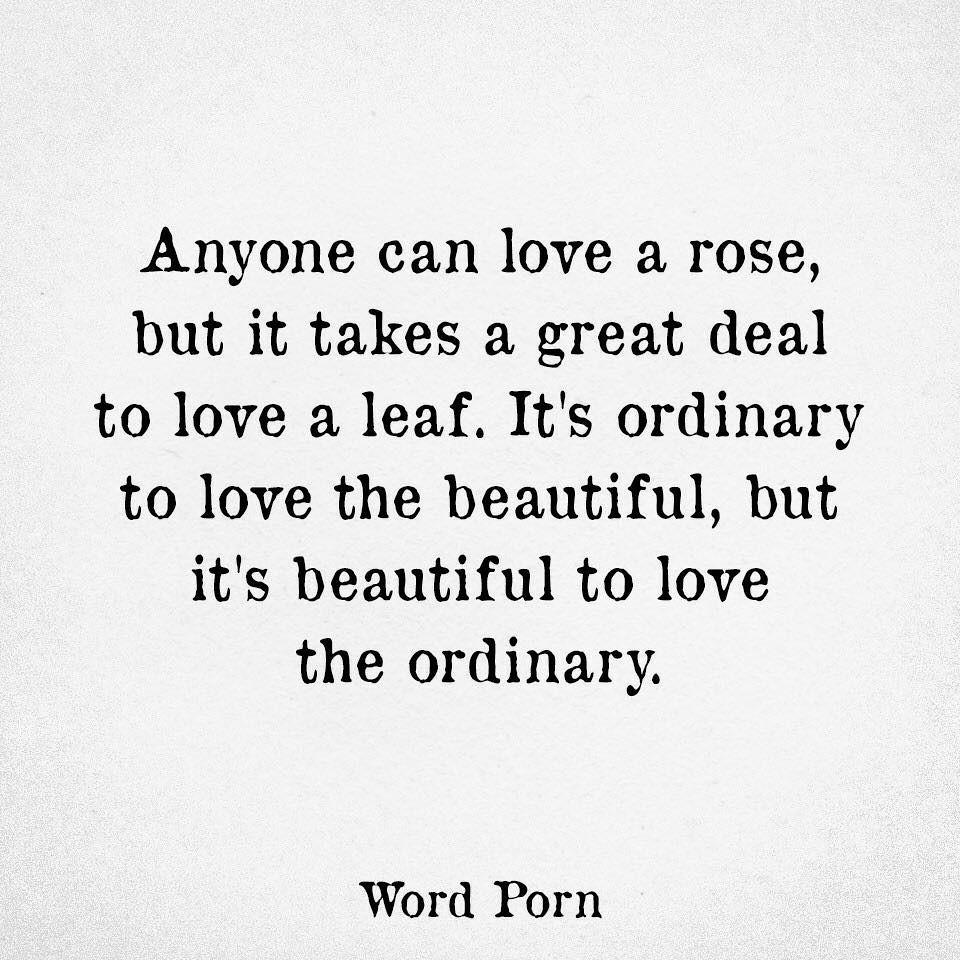In the image, a poetic inscription is rendered in bold black ink on a light gray background. The text reads: "Anyone can love a rose, but it takes a great deal to love a leaf. It's ordinary to love the beautiful, but it's beautiful to love the ordinary." The phrase "Word Porn" is centered at the bottom, with both the "W" and "P" capitalized. The lettering follows standard capitalization and punctuation rules, enhancing the visual appeal of the quote against the subtly colored backdrop.